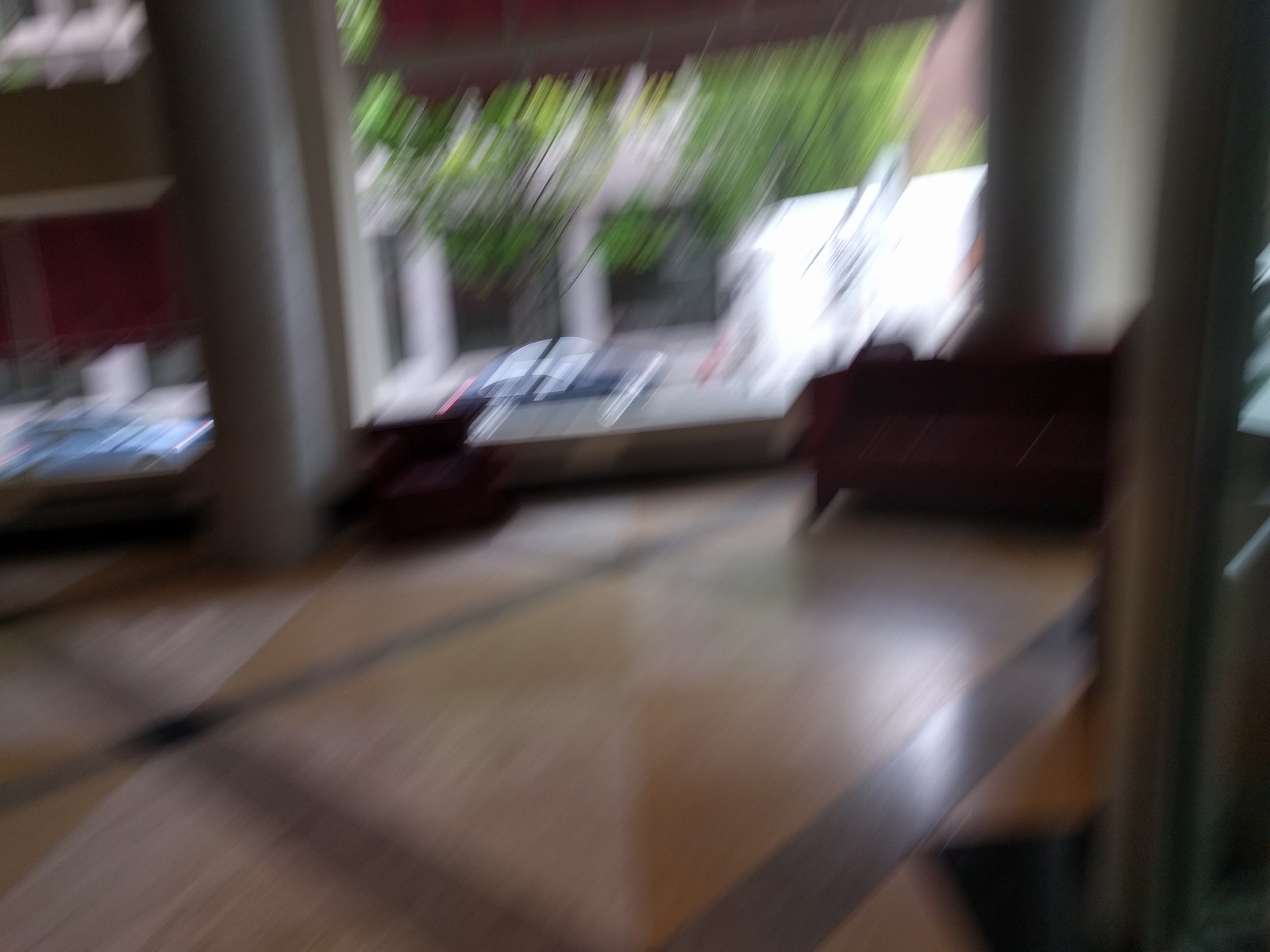This image depicts a commercial space viewed from the inside, with the scene unfolding through a large window that captures the bustling street outside. The wide, blurry, and out-of-focus frame makes it challenging to discern specific details, but various elements are still identifiable. On the left side of the image, a blue car appears to be moving rightward, while another car, possibly heading in the opposite direction, is partially visible. Additionally, a white van is also seen on the street. A tree and the windows of a store across the street are noticeable in the background.

Inside the space from which this scene is viewed, the floor is covered in large orange tiles bordered by a darker color, with light reflecting off the surface, adding to the overall ambiance. Two columns, potentially serving as window frames, divide the view. Various indistinct objects occupy the interior space, though they remain unclear due to the image's underexposure and blurriness. Despite the lack of sharpness, the composition suggests an active urban environment just beyond the windowed facade.